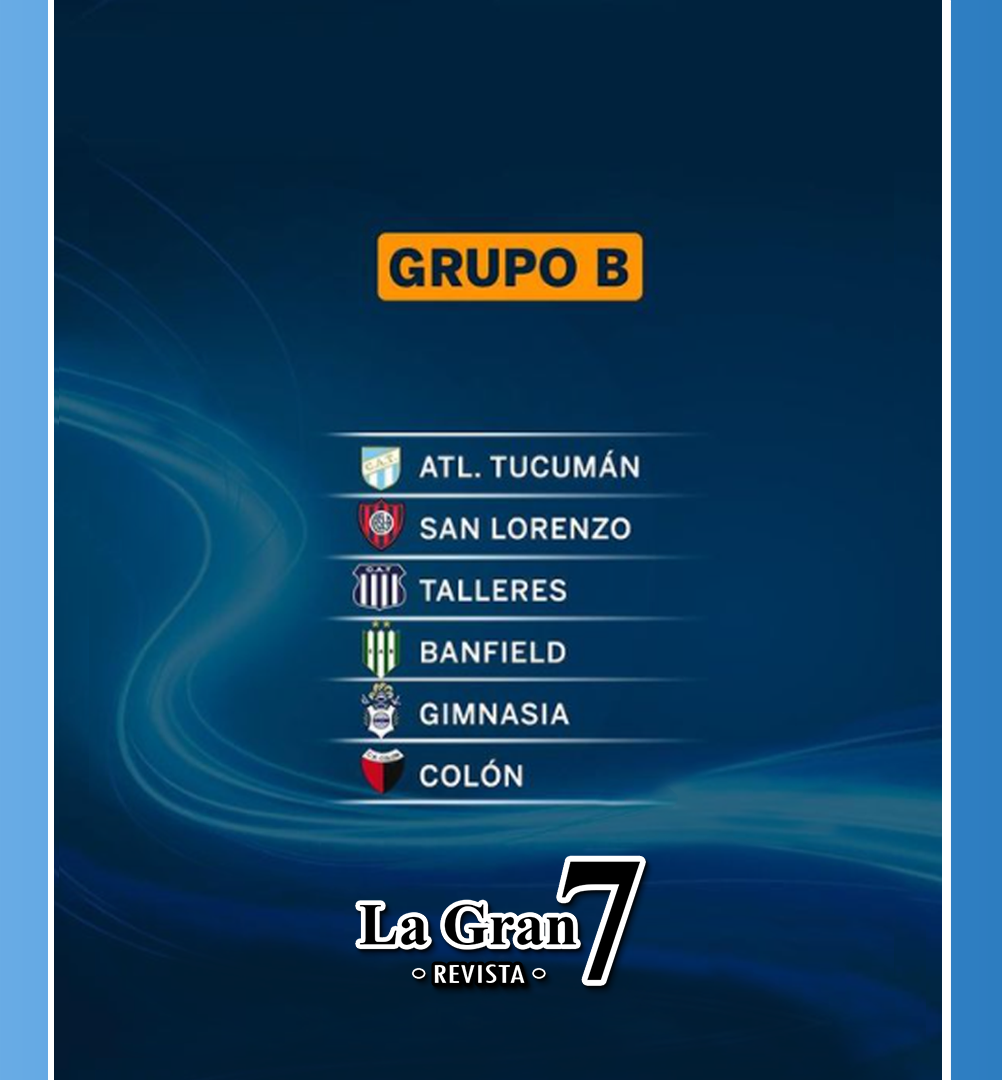The image is a promotional poster for various sports teams, characterized by a dark navy blue background and accentuated by light blue lines and swirls. There are two prominent light blue vertical rectangles running from top to bottom on each side of the poster. Across the top center, an orange rectangle with rounded corners features the text "GRUPO B" in black letters. Below this, white lines separate different team information, listed one beneath another.

The first team displayed is "ATL Tucumán," with its crest on the left in blue and white with a cream color, featuring a symbol over the A and N. Next, separated by another light blue line fading into dark blue, is "San Lorenzo," identified by a red and black striped shield with a white circle in the middle. Following is a blue and white shield for "TALARS." 

Then comes "Banfield," represented by a blue and green shield. Next is "Gimnasia," with a shield featuring blue edges and a brown top. Finally, "Colón" is shown with a red and black shield topped in white. At the bottom, the text "La Grande 7 Revista" stands out in large black letters outlined in white, emphasizing the grand nature of the presentation.